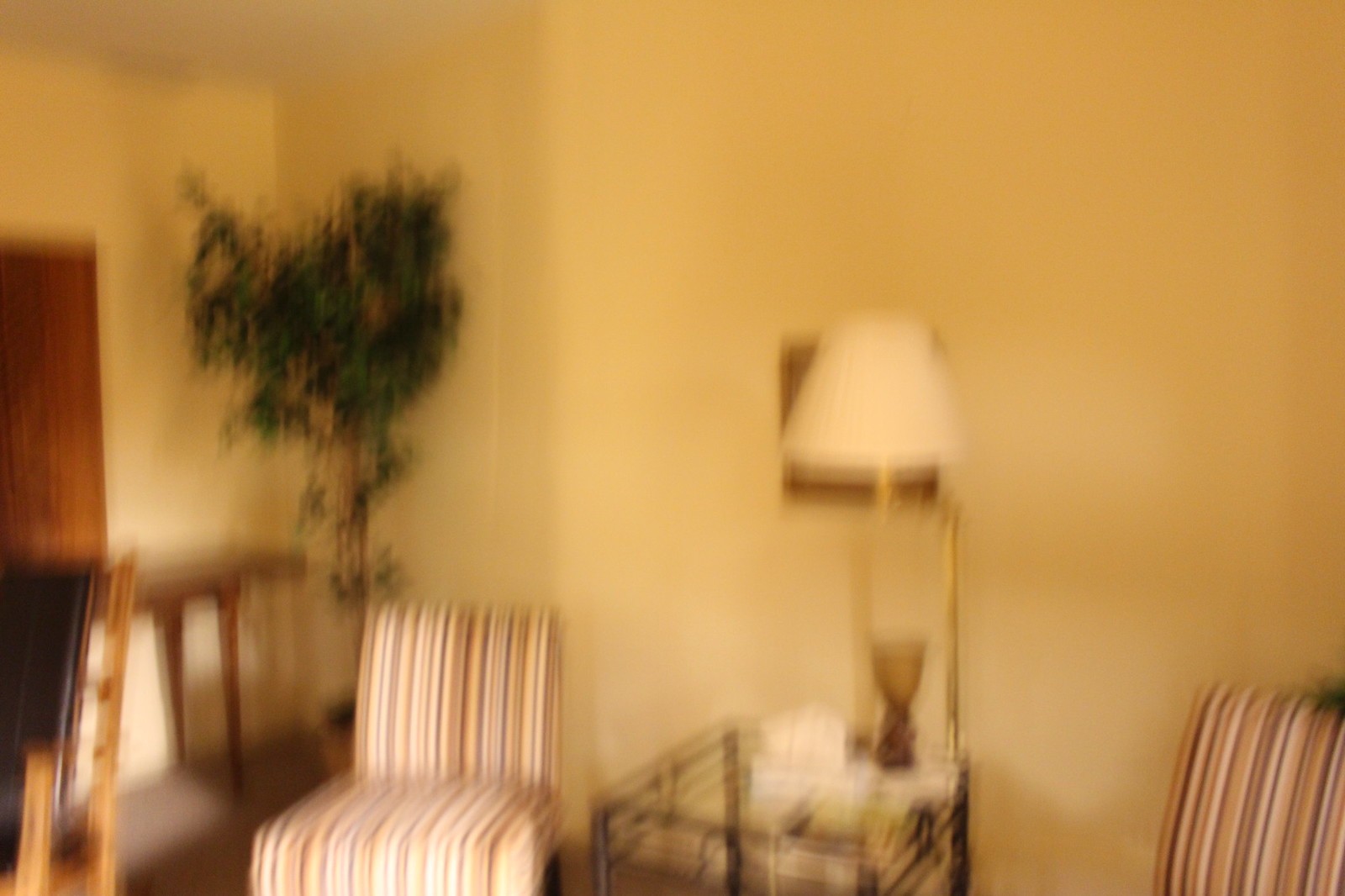This indoor, horizontal image taken in a residential area is noticeably blurred and has a predominant yellowish-orange tint. The scene features a pair of armless chairs with vertically striped upholstery flanking a glass-top end table. Atop the table sits a tall lamp with a white shade, which partially obscures a framed object behind it. The background walls exhibit a similar yellowish-orange hue, although their original color might be white. In the left corner of the room, a small tree stands next to a brown table and a chair with black leather-like upholstery. A plain brown door is centered along the left side of the room, enhancing the cozy, albeit slightly cluttered, interior.